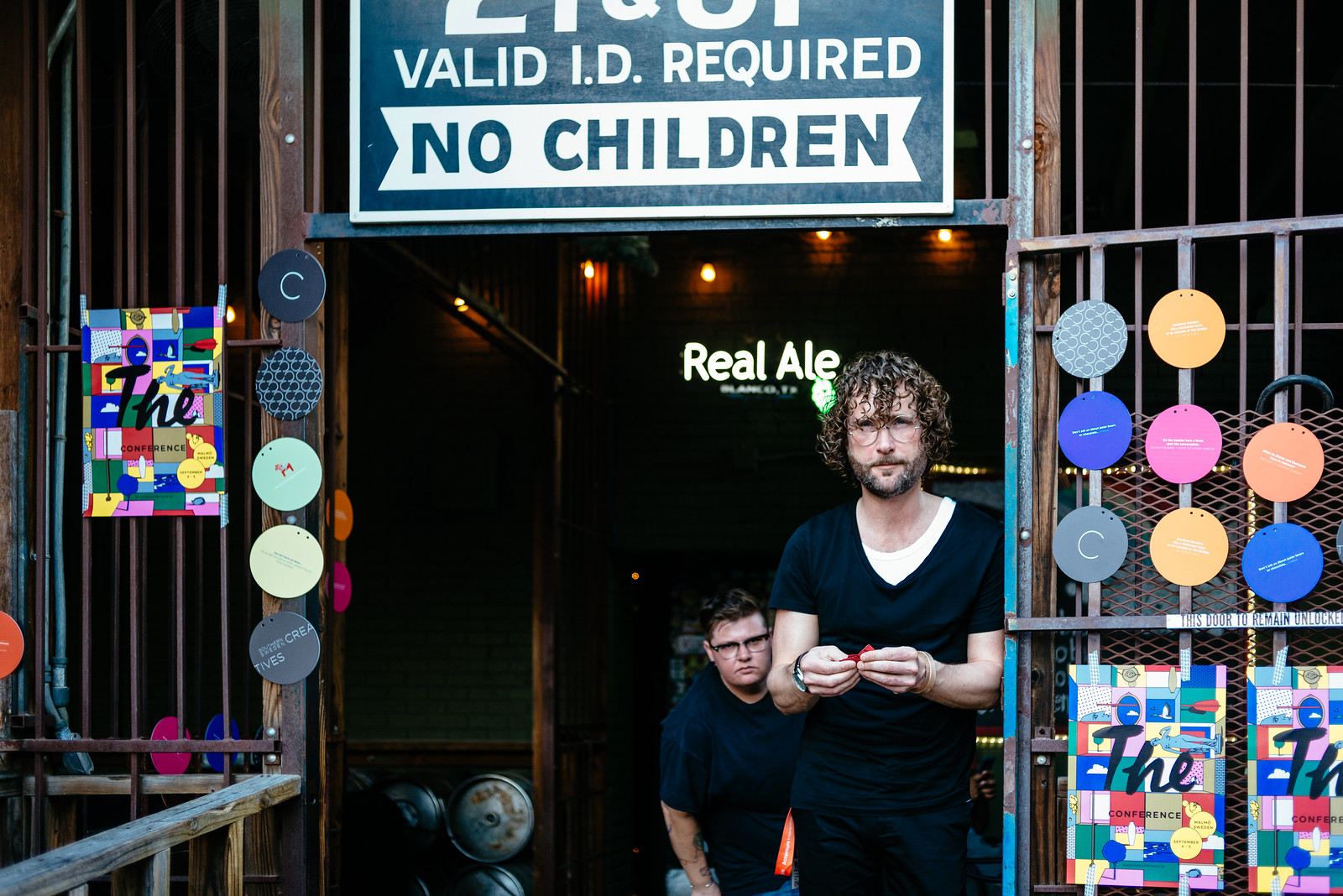This vibrant photograph depicts the entrance to a bar or event venue with strict age restrictions, as indicated by the prominent sign reading "21 and up, valid ID required, no children" displayed in shades of blue and white at the top of the doorway, framed by metallic bars reminiscent of a security door. At the center of the image are two men; the one in the foreground, with curly hair, glasses, and a beard, is dressed in a dark V-neck t-shirt over a white tank top and holds a ticket, suggesting he manages admissions. Above his head, a sign reads "REAL ALE," hinting at the sale of craft beers inside. Behind him, standing at elbow height, implying a possible descent of steps, is another man with shorter dark hair and glasses, who looks less pleased. Both men are framed by a collage of colorful coasters and geometrical papers taped to the doorframe, adding a quirky and vibrant atmosphere. A multicolored sign with the words "THE CONFERENCE" in large black letters on the left side further complements the eclectic decor.